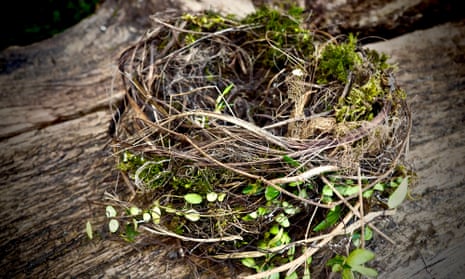This detailed close-up photo showcases a bird's nest intricately crafted from various materials. The nest, appearing to be about 20 inches in diameter and rising approximately 15 inches high, is perched centrally on a raw wooden log with uneven dark and light splotches, resembling driftwood. The nest itself is tightly wrapped with branches and twigs of varying shades of brown and interspersed with forest green leaves, some of which poke out from the front and back. Among the twigs and leaves, there's a mix of long brown grasses, leafy reeds, and yellowish-beige leaves, creating a rich texture. The top of the nest is thoughtfully adorned with additional green leaves, some moss, and scattered feathers, contributing to its natural depth. In the background, dark, out-of-focus leaves can be seen in the left-hand corner, adding to the scene's organic feel. The photograph captures the nest during the day, emphasizing the detailed craftsmanship intended to attract attention.